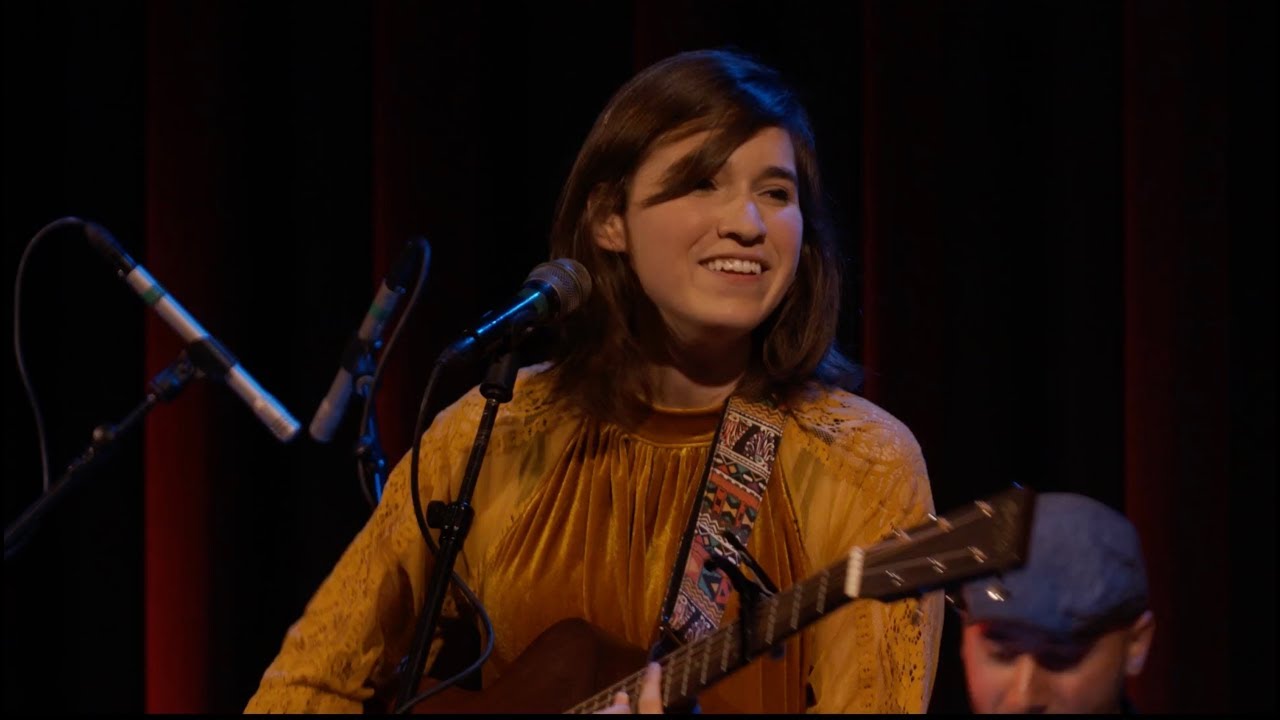This horizontally rectangular, full-color photograph captures an indoor musical performance featuring a young caucasian woman as the main focus. She has shoulder-length, straight brown hair with side-swept bangs, and some of her hair partially covers one eye. She is dressed in a tan felt or velour top and holding an acoustic guitar with a multicolored strap. The image shows her from chest up, and she is looking slightly to the right with a subtle grin on her face. She is standing at a microphone, with another microphone visible to her left. The background consists of blackness interspersed with folds of red curtains, dimly lit by artificial lighting. In the bottom right corner, there is a caucasian man wearing a blue or denim newsboy cap, looking downward. The color palette of the photo includes black, gray, orange, yellow, red, brown, tan, and silver, emphasizing the subdued indoor lighting.